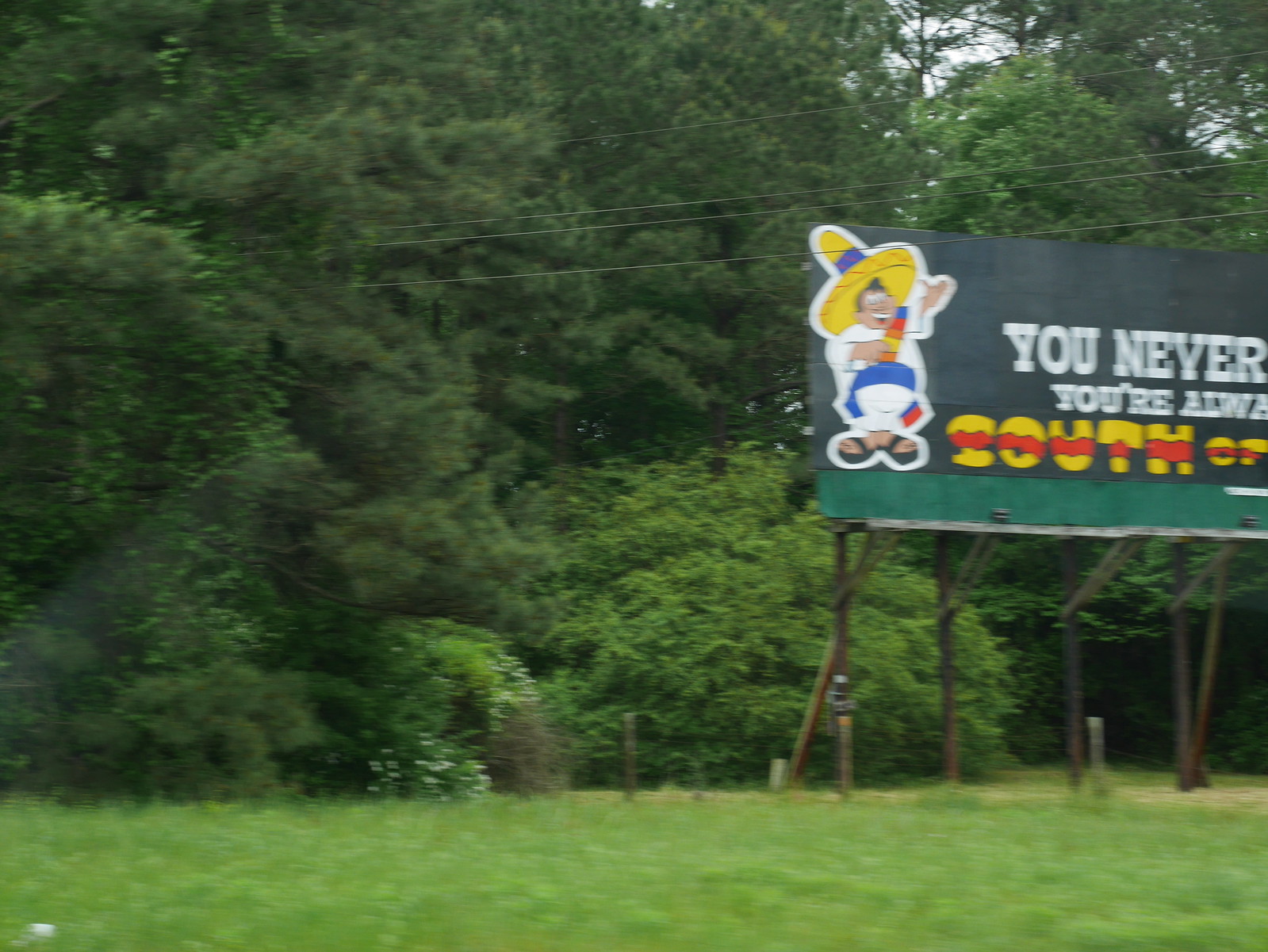Captured during the day, this photograph showcases a grassy area stretching horizontally across the bottom portion of the image. Beyond the grass, a wire fence with a visible wooden post extends from the center to the right, though the wire itself is faint and partially obscured. Dominating the right side of the image is a large billboard sign, with only the left half visible. The billboard features an illustration of a Mexican man wearing a large sombrero, a white outfit adorned with blue and red accents, and black sandals. Below the figure, the text "South of" is legible, though the rest is cut off, making the full message unclear. The backdrop of the image is composed entirely of dense trees, leaves, and bushes, leaving no glimpse of the sky.